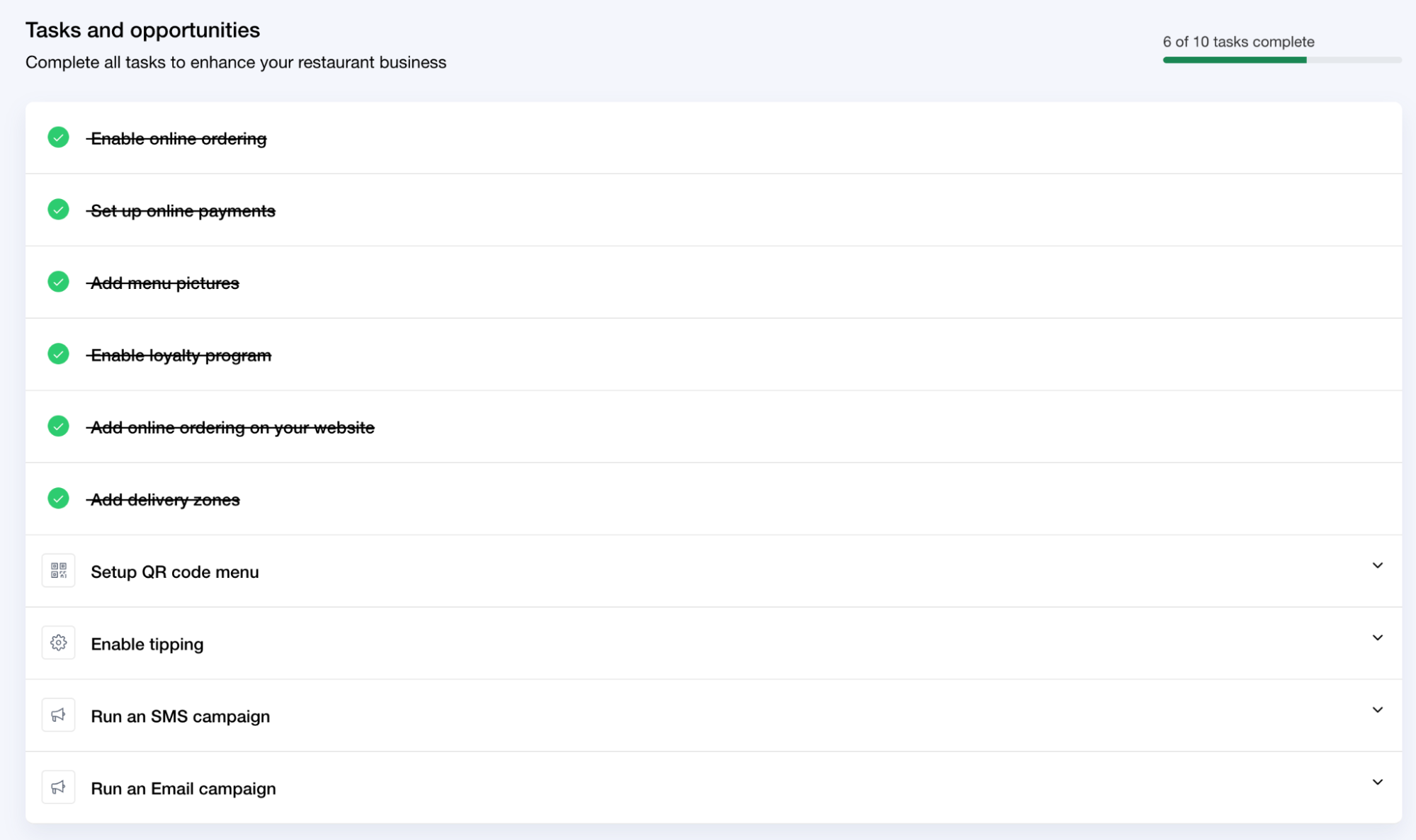The image depicts a screenshot of a "Tasks and Opportunities" menu designed to help enhance a restaurant business's operations. The background is predominantly white, framed by a light gray border with a gray bar running across the top. The top bar prominently displays the title "Tasks and Opportunities" in black text, accompanied by the directive "Complete all tasks to enhance your restaurant business and operate." Below the title, a progress bar shows that six out of ten tasks have been completed, with the progress visually indicated by a partially filled green bar.

The menu lists ten tasks in total, arranged in ten rows. The first six tasks have been successfully completed, each marked with a green checkmark and struck through with a horizontal line. These tasks include:

1. Enable online ordering
2. Set up online payments
3. Add menu pictures
4. Enable loyalty program
5. Add online ordering on your website
6. Add delivery zones

The remaining four tasks, which are yet to be completed, are listed as follows:

7. Set up QR code menu
8. Enable tipping
9. Run an SMS campaign
10. Run an email campaign

Each incomplete task is written in standard black text, without any strike-through or checkmark.